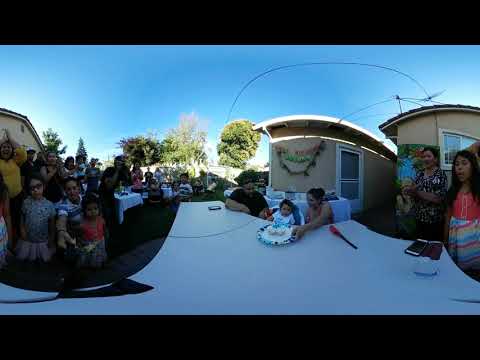In this vibrant image of a backyard birthday party, it appears to be a celebratory gathering for a young child's birthday, possibly their first. The focal point of the scene is a white table at the center where a family—comprising a mother, father, and their young child, potentially in a high chair—are seated, presenting a cake to the child. The table, slightly curved and distorted due to the panoramic shot, holds a plate with a piece of cake and candles, alongside a lighter used for lighting the candles. Surrounding the table are numerous family members and friends, all gathered to sing happy birthday and share in the joyous moment. The background features ranch-style houses closely set together amidst green trees, adding to the serene suburban atmosphere. The bright, sunny day illuminates the colorful decorations on the house behind them and highlights the festive spirit of the occasion.